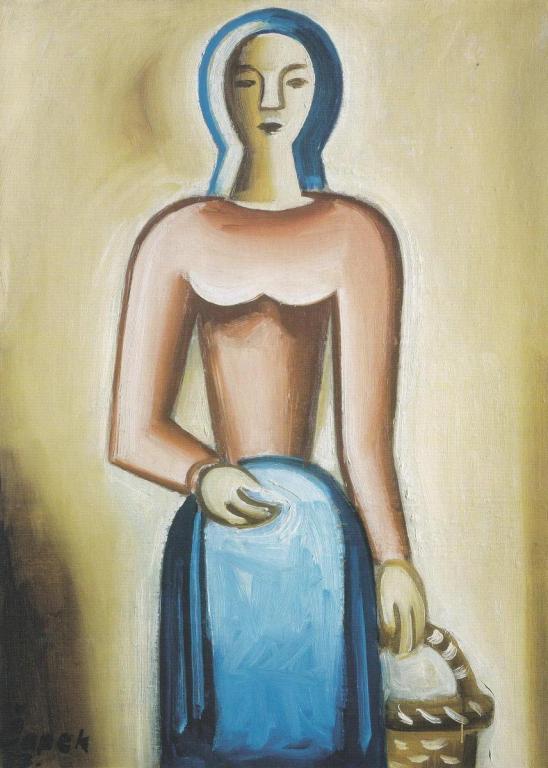In this Expressionist and Cubist-influenced painting titled "Devce S. Koshem" by Joseph Capek, created in 1923, a young woman is depicted using basic geometrical shapes and a palette of beige and blue. The woman stands facing the viewer, with her blue hair framing her face, which features a prominently large nose. She wears a long-sleeve beige or brown top and a loose, flowing blue skirt. Her left hand holds a golden wicker basket near the bottom of the painting, while her right hand is bent, resting on her belly. The background consists of painterly beige tones, enhancing the stylized and abstract nature of the artwork.